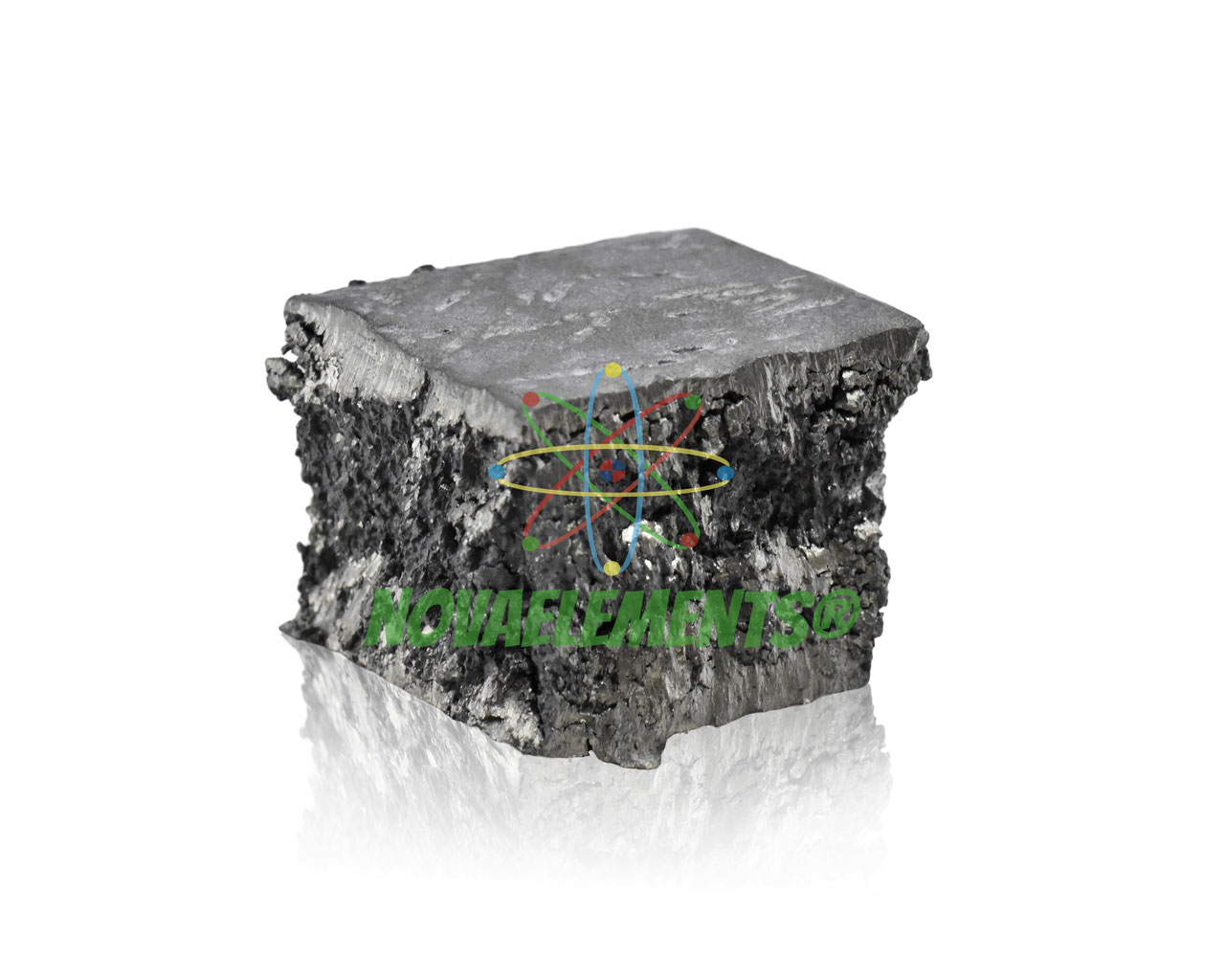The image showcases a three-dimensional close-up of a metal block with a white background. The top of the metal is a thick, unevenly cut cube, featuring a generally smooth surface interspersed with rough patches. The middle part of the block is extremely rough and textured, resembling the craggy side of a cliff with a mix of light gray, dark gray, and medium gray tones. The bottom and front of the block return to a mostly smooth surface, though they still possess occasional bumps. Superimposed on the surface of the metal is a watermark, displaying the large green text "NOVA Elements®". Additionally, the image features several intersecting atom-like circles in varied colors: yellow, blue, green, and red, each composed of a single dot at the end of each circle. Shadowing beneath the metal block adds depth to the image.